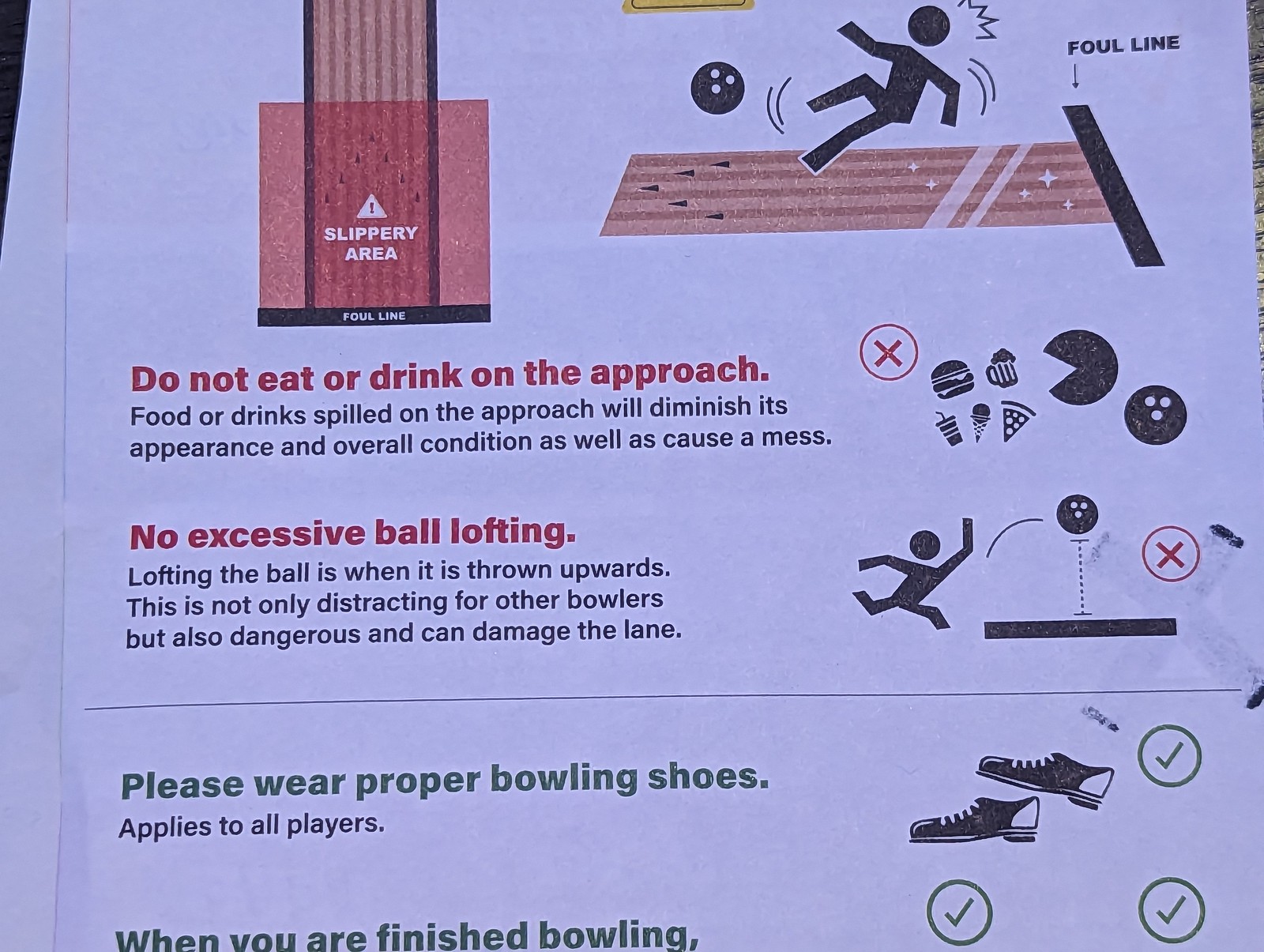This image features a safety and instructional poster likely placed in a bowling alley. The background is a light purple, and the poster is filled with black, red, and green text alongside illustrations. At the top left, there is a warning sign in red that says "Slippery Area" with an exclamation point, and below it explains, “Do not eat or drink on the approach,” emphasizing that spills can diminish the alley’s appearance and condition, as well as cause messes. Next, in red text, it states “No excessive ball lofting,” further explained in black text that lofting—throwing the ball upwards—not only distracts other bowlers but can also be dangerous and damage the lane, accompanied by an illustration demonstrating this. Finally, in green text, the poster advises, “Please wear proper bowling shoes,” applicable to all players, highlighted by an illustration of black bowling shoes. This comprehensive guide is designed to help maintain safety and proper etiquette in the bowling alley.